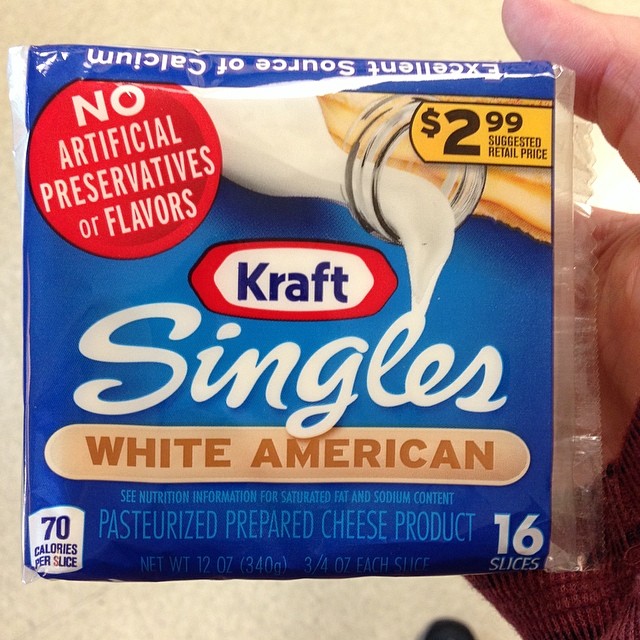This is a square-shaped photograph of a package of Kraft Singles cheese slices. A hand, with the palm facing the viewer and the thumb positioned at the top, holds the package, likely supported by the index and middle fingers. The background is a beige, tile-like surface, possibly a kitchen wall, in a tan-yellow shade. The Kraft Singles package dominates the image and is slightly off-center to the left. The plastic wrapping of the cheese slices is predominantly blue and features multiple labels and copy. A prominent red circle declares "No Artificial Preservatives or Flavors." The Kraft logo is clearly visible, as is the word "Singles." Additionally, an image of a glass jar of milk pouring into the word "Singles" is included, emphasizing the cheese's dairy content. The text "White American" is highlighted within an oval, and "16 Slices" is noted in the lower right-hand corner.